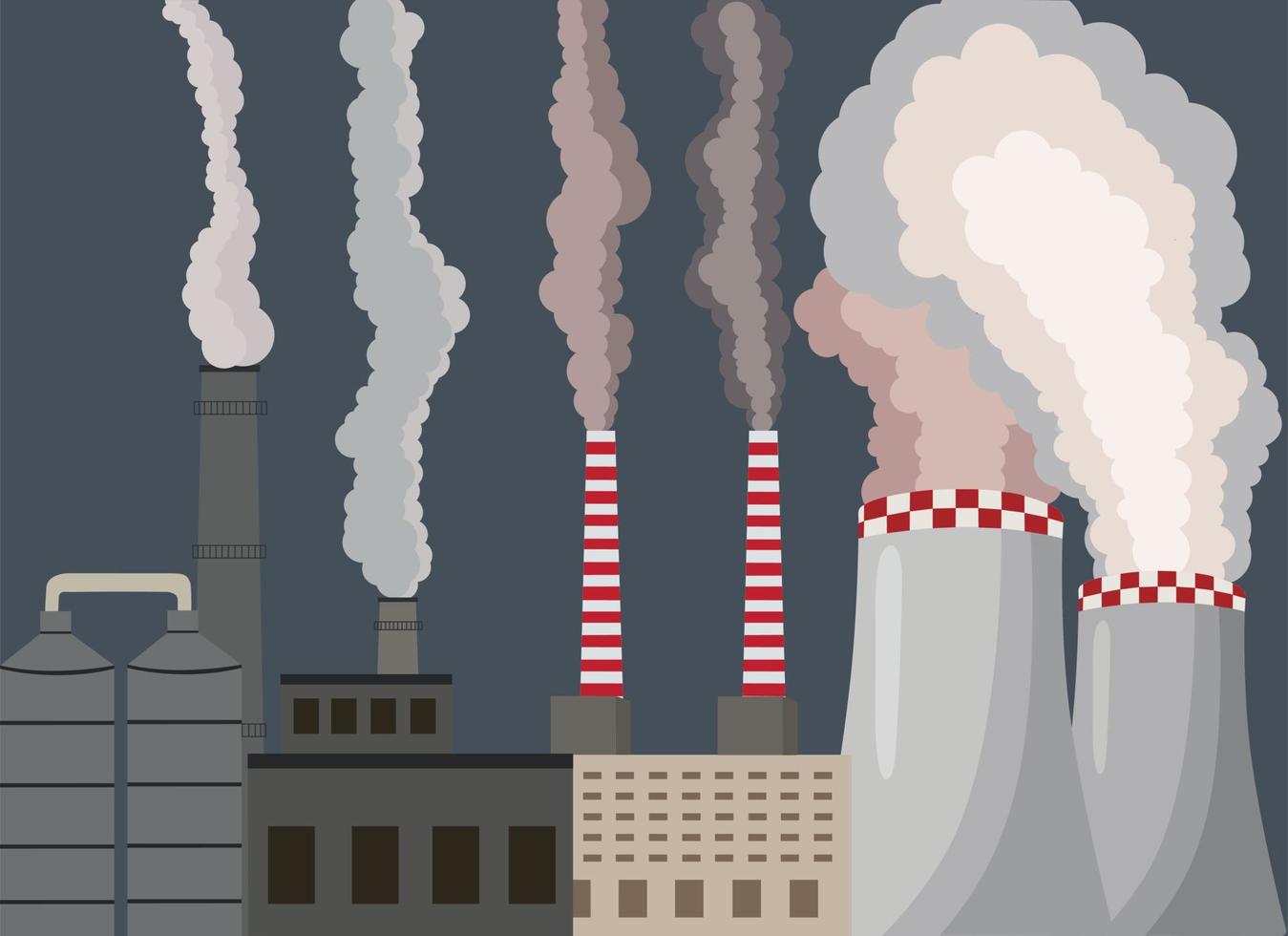This is a minimalistic, computer-generated illustration depicting an industrial landscape with various factories and smokestacks emitting smoke into a dark gray sky. There are approximately six smokestacks, including two that resemble nuclear reactors and are striped in red and white. The smoke varies in color, including shades of white, red, gray, and pink. The simplistic design, reminiscent of a 2D chart or infographic, emphasizes the emissions from these industrial sites and highlights the environmental impact visually.